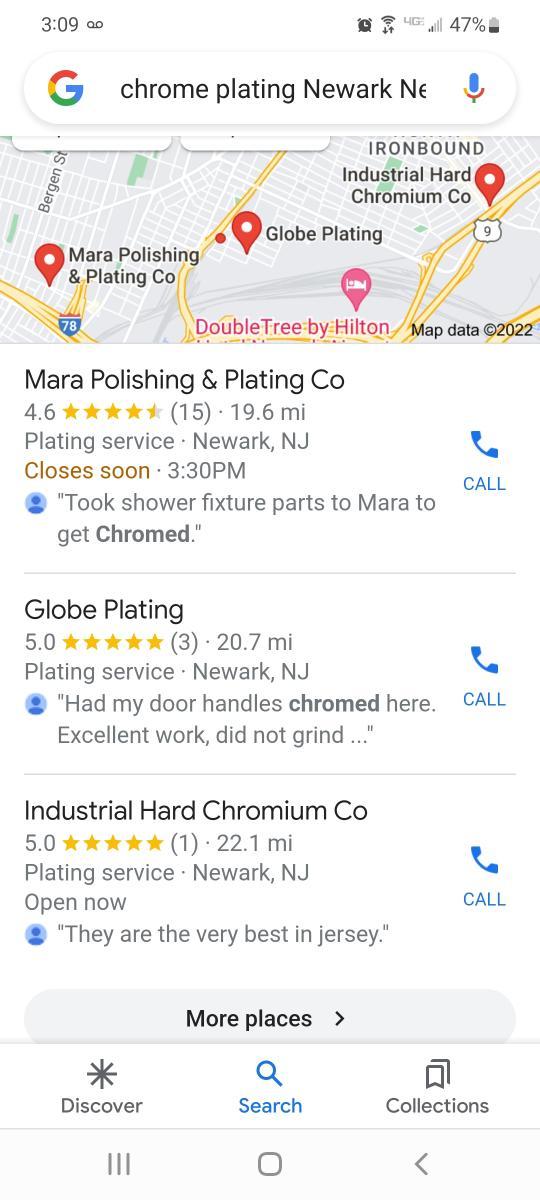The image displays a screenshot from a phone or tablet, evident from the status bar at the top showing the time as 3:09, along with various icons including a voice recording symbol, a clock, a Wi-Fi signal indicator, a 4G data symbol, and a battery at 47%. Below this, the screenshot captures a Google Chrome browser page where the user has searched for "chrome plating new work," presumed to be in New Jersey. 

The search results feature a map highlighting three main establishments: 
1. **Mirror Polishing and Plating Co.**, rated 4.6 stars from 15 reviews and located 19.6 miles away.
2. **Globe Plating**, boasting a 5-star rating from 3 reviews, situated 20.7 miles away.
3. **Industrial Hard Chromium Company**, also with a 5-star rating from a single review, found 22.1 miles away.

Next to each establishment’s details, there is a call button for easy contact. Further down the page, there is a "More places" button for additional options. At the bottom of the screen, navigation tabs for "Discover," "Search," and "Collections" are visible.